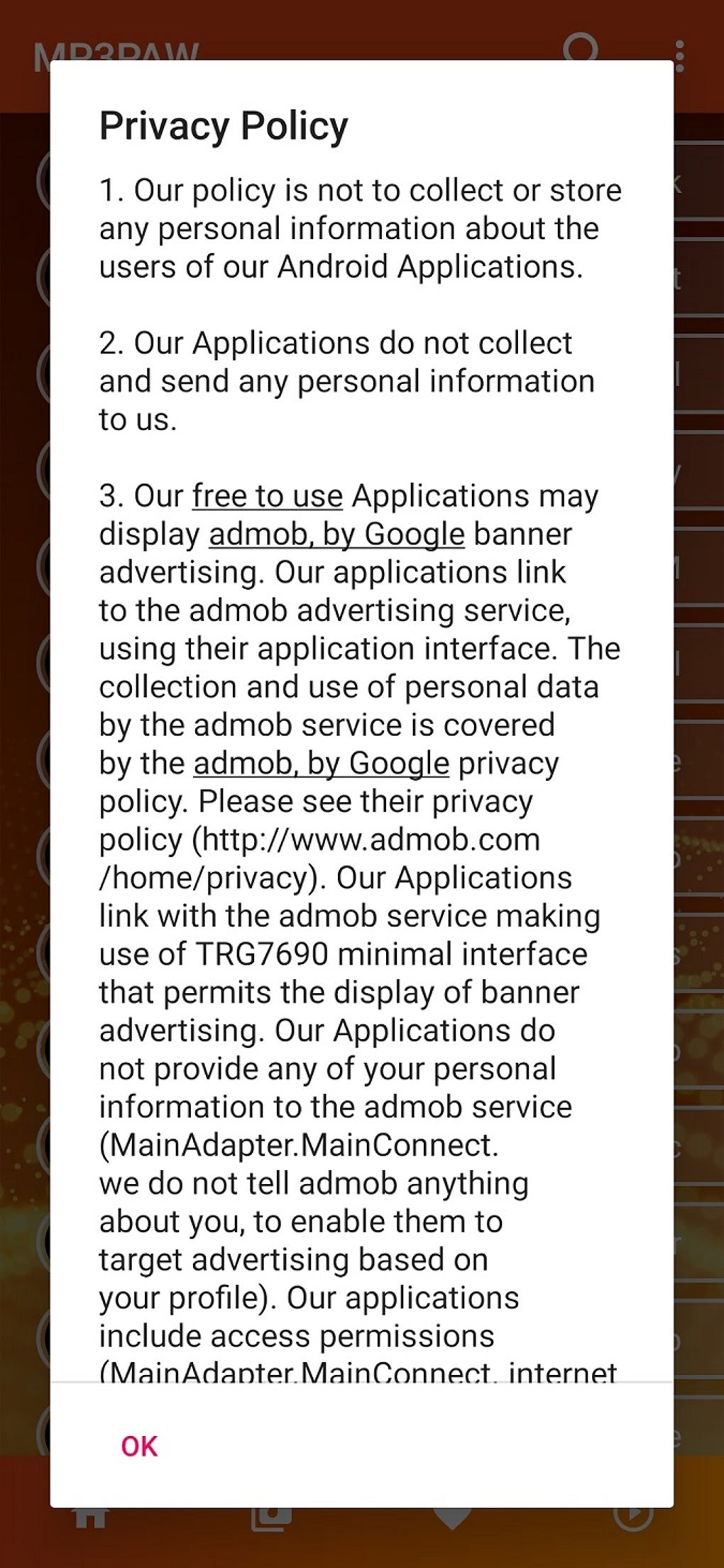The image showcases a Privacy Policy displayed on a smartphone screen, with the policy text superimposed over an orange and brown background. The privacy policy is presented within a large white, vertically oriented rectangle, featuring black text. At the top left, the title "Privacy Policy" is prominently displayed in bold. The policy outlines several key points:

1. The policy asserts that it does not collect or store any personal information about users of their Android applications.
2. It confirms that the applications do not collect or send any personal information to the developers.
3. The policy mentions that their free-to-use applications may display AdMob by Google Banner advertising. These applications link to the AdMob advertising service via their application interface, and the collection and use of personal data by AdMob is governed by the AdMob by Google Privacy Policy, which can be found at http://www.admob.com/home/privacy.

Furthermore, the text explains that the applications connect with the AdMob service utilizing the TRG7690 minimal interface to display Banner advertising, without providing any user personal information to AdMob. The policy reiterates that the developers do not share user data with AdMob for targeted advertising purposes. Additionally, the applications include access permissions such as "mainadapter.mainconnect.internet."